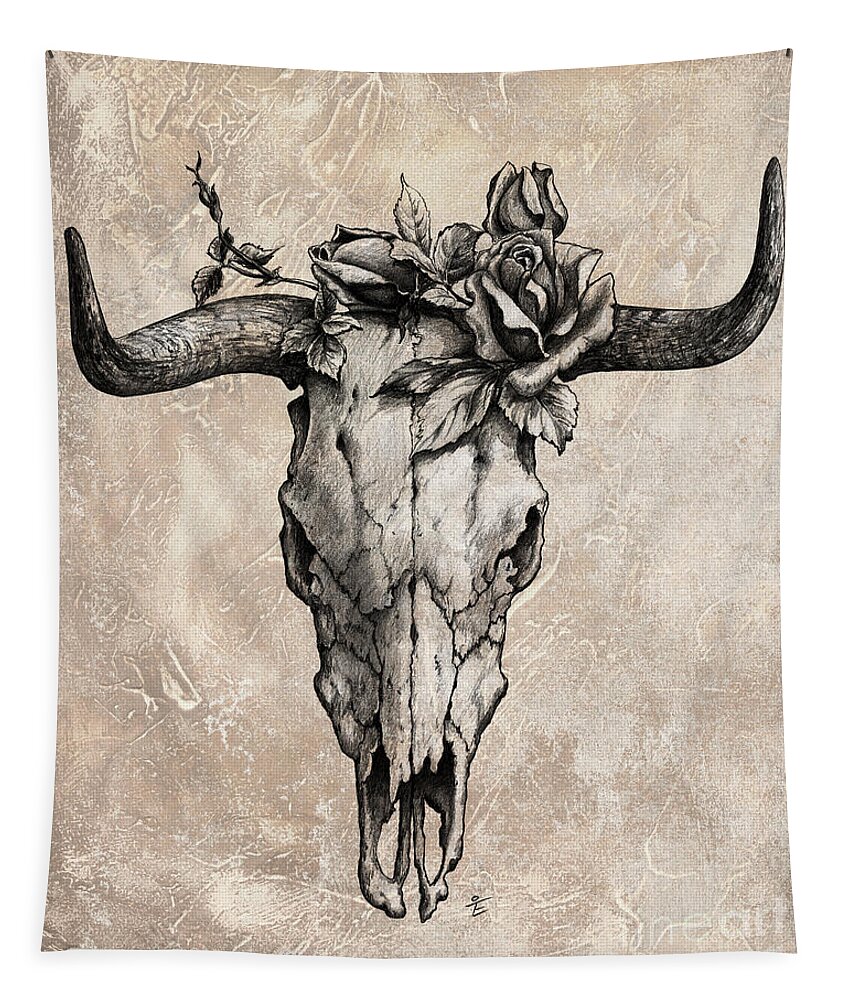The image depicts a detailed drawing of an ox or bull skull facing directly at the viewer. The skull, adorned with large horns on either side, is characterized by a significant break at its nose and prominent eye sockets. A long vertical line runs down the center of the skull. Atop the skull and slightly to the right, several wilted flowers, including what appears to be a rose, are intertwined with a curving stem and a few leaves. The artwork, rendered in black and white with possible charcoal or pencil, sits on an aged, off-white canvas with a gray, marble-like texture that suggests it may be leather. The canvas appears tattered and stretched at the corners, giving it a worn, historical look. At the bottom right, a faded watermark reads "N-E-A-L-T," though it's partially obscured. The overall aesthetic bears a resemblance to a Georgia O'Keeffe painting.